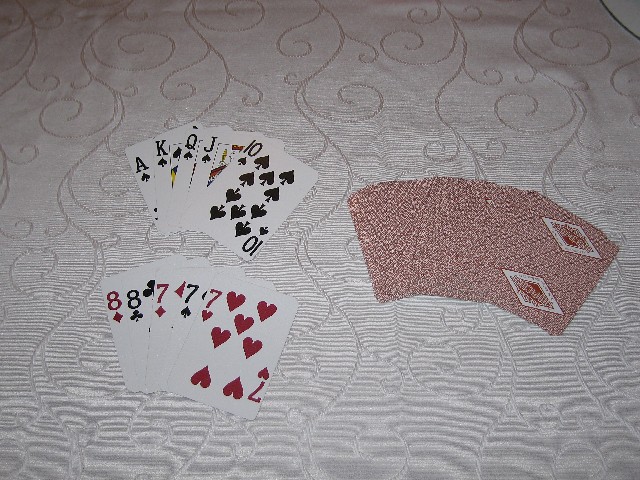This photograph captures a meticulously arranged scene featuring a pristine white tablecloth adorned with subtle, curling line patterns resembling vines and intersected by horizontal white stripes. Positioned strategically on the tablecloth are three distinct stacks of playing cards. To the left, there are two stacks: the upper stack showcases the faces of the Ace of Spades, King of Spades, Queen of Spades, Jack of Spades, and Ten of Spades, with the Ten of Spades prominently displayed on top. Below this, another fan of cards reveals the Eight of Diamonds, Eight of Clubs, Seven of Diamonds, Seven of Spades, and Seven of Hearts. On the right side of the table, approximately ten playing cards are fanned out, displaying their uniform backs. The careful arrangement and clarity of each card's position make this photograph both visually captivating and rich in detail.